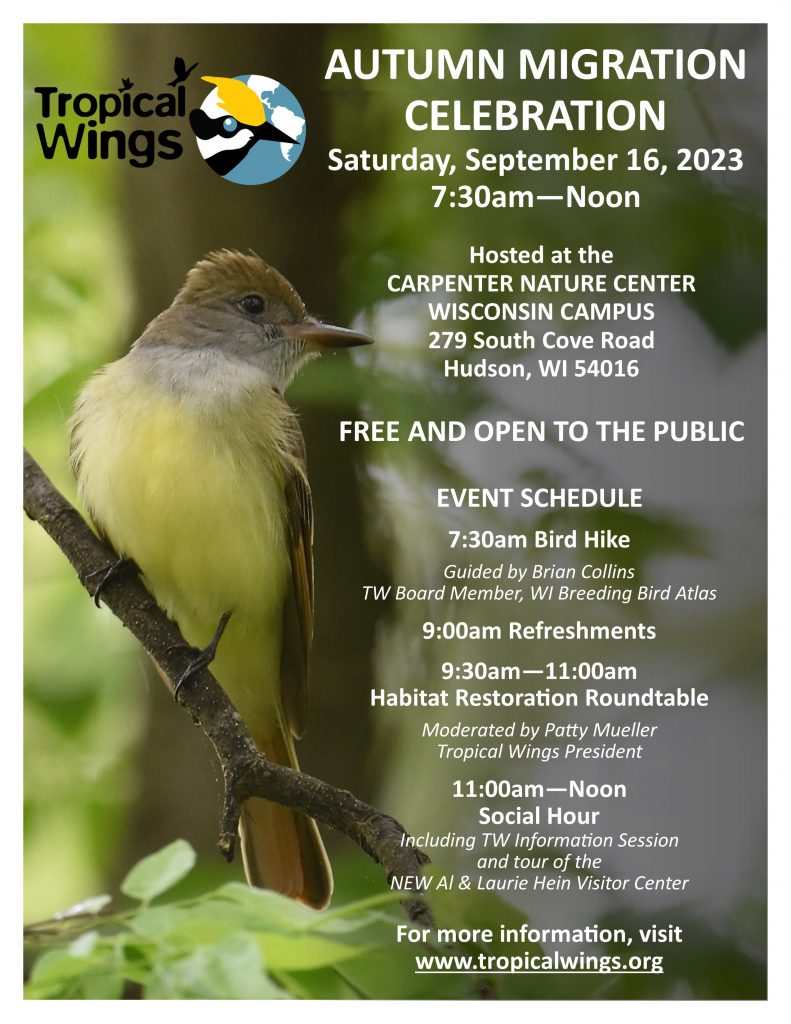This bright green event poster features detailed artwork of a bird positioned to the left. The bird has a white body with a greenish-brown head, a brown neck, and dark legs wrapped around a brown branch, set against a backdrop of a leafy green tree. At the top of the poster, "Tropical Wings" is prominently displayed in black font alongside a logo of a bird's head encircled. The main text, in white font, advertises the "Autumn Migration Celebration" occurring on Saturday, September 16th, 2023, from 7:30 a.m. to noon at the Carpenter Nature Center, Wisconsin Campus, located at 279 South Cove Road, Hudson, Wisconsin, 54016. The event is free and open to the public. The schedule includes a 7:30 a.m. bird hike guided by Breon Collins, a 9 a.m. refreshment break, a habitat restoration roundtable from 9:30 a.m. to 11 a.m. moderated by Patti Mueller, and an 11 a.m. to noon social hour along with a tour of the new Al and Lori Hine Visitor Center. For additional information, attendees are directed to visit www.tropicalwings.org. The poster emphasizes its appeal to bird watchers and nature enthusiasts, highlighting activities around birding and habitat conservation.